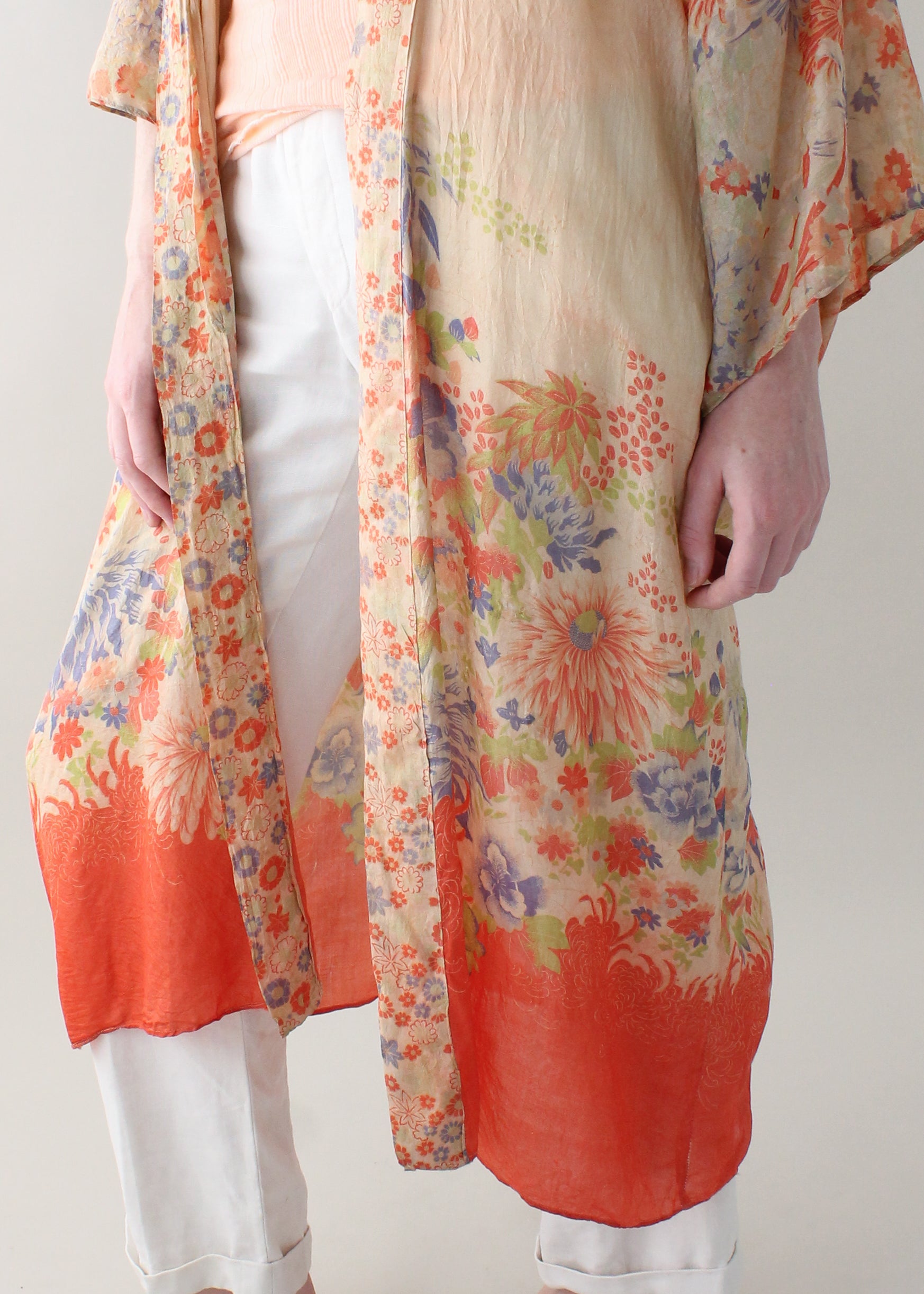In the photo, we see the bottom half of a woman, identifiable as white by her hands, modeling an eclectic outfit. She is wearing a lightweight, open-front kimono-style cardigan that falls to about her knees. The cardigan has a peach and beige base color with a vibrant floral pattern featuring orange and blue flowers placed near the sleeves and the hem. The hem also sports a solid dark orange band. She pairs this with a tucked-in peach short-sleeved shirt and white pants with cuffs at the bottom. The image captures her from a little above the waist down to her ankles, with her arms hanging naturally by her sides. The entire ensemble is presented in a way that showcases the unique details and flow of the cardigan.